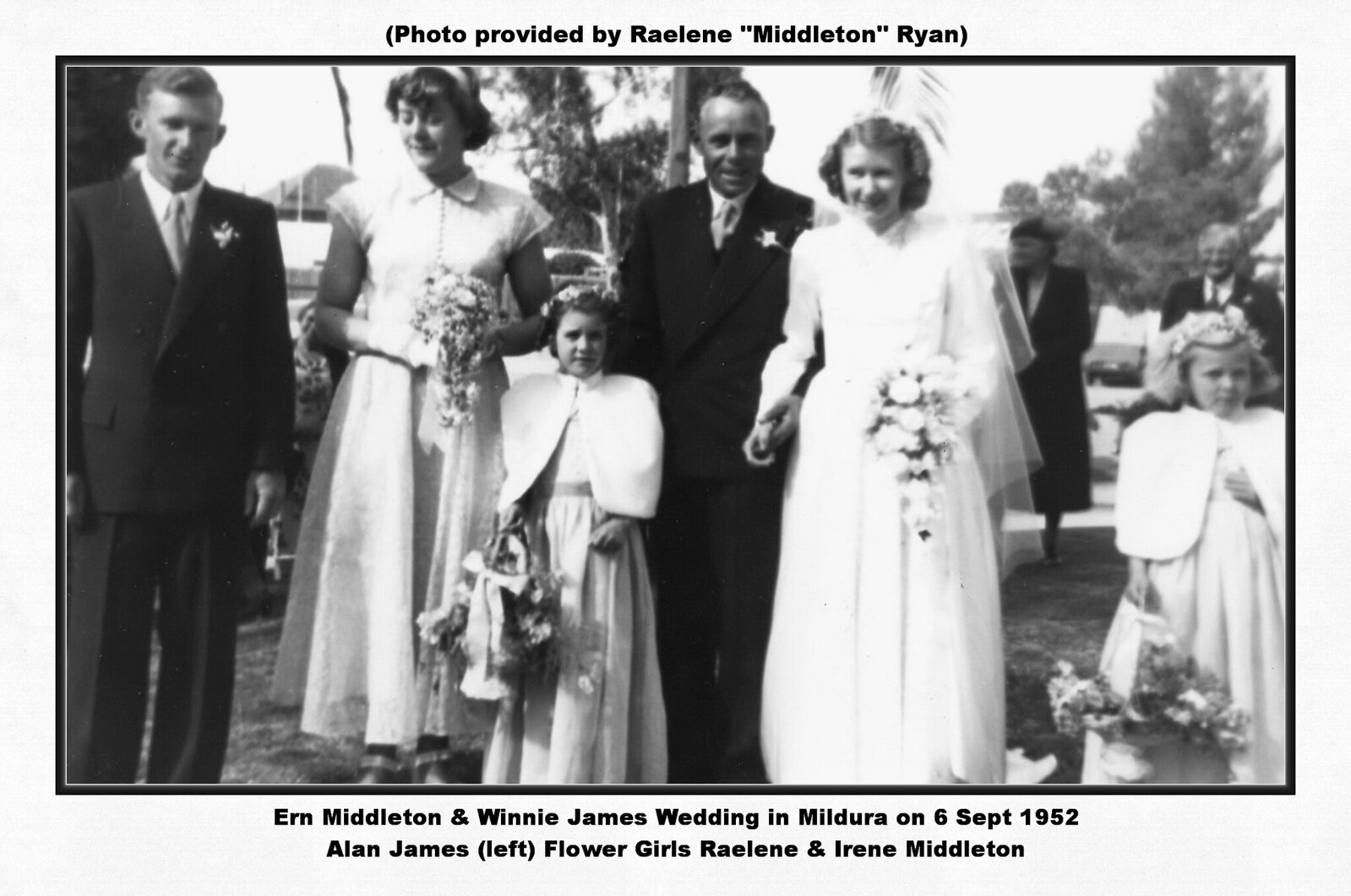In a black and white photograph surrounded by a thick gray border with an inner thin gray border forming a frame, the text at the top reads "Photo provided by Berlin Middleton Ryan." The text at the bottom states, "Ern Middleton and Winnie James wedding in Mildura on 6th September 1952. Alan James left flower girls Raleen and Irene Middleton."

The image captures a moment from their wedding day with multiple people facing forward. On the far left stands a man in a black, buttoned suit with a floral arrangement on his lapel. He is wearing a white shirt and a tie. Next to him is a woman in a short-sleeve, light-colored dress, holding a bouquet of flowers. She is followed by a young girl, around seven years old, in a long dress with a cape around her shoulders, holding a basket of flowers in her left hand. 

Further to the right is another man in a two-piece suit, possibly holding the hand of a bride dressed in a long-sleeve, white dress and holding a bouquet of flowers. Beside the bride stands another young girl, similarly dressed in a long dress with a cape, holding a basket of flowers. Trees can be seen in the background, indicating that the photograph was taken outside, with a few other people standing behind the main subjects.